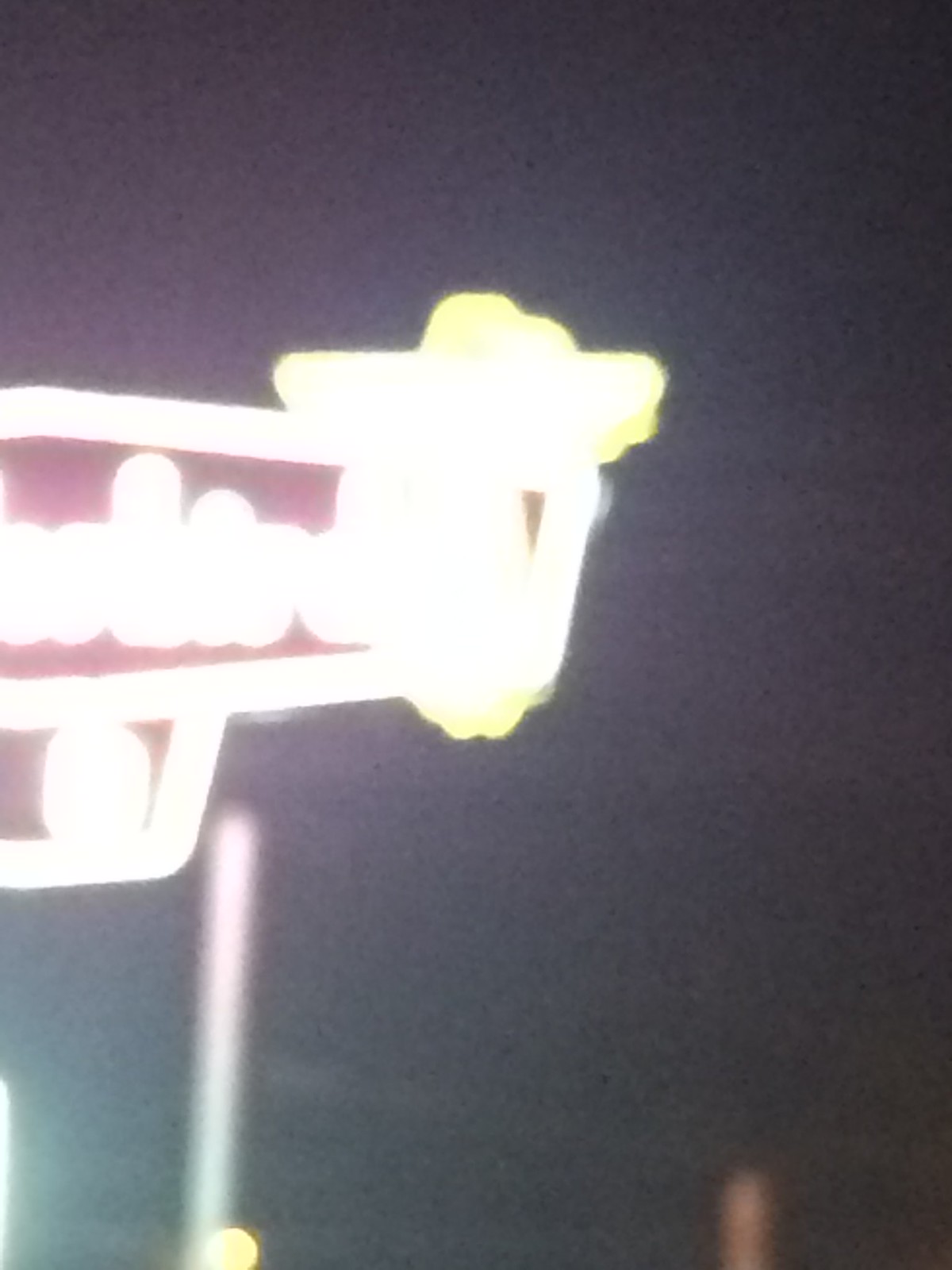The image appears to depict a neon sign, likely belonging to a restaurant or similar establishment. The sign is extremely bright, making it difficult to read the text, especially on the right side where the light is overblown. The illuminated text is enclosed in a box-like area, and next to this text on the right side, there is a symbol resembling an angel. This angel-like figure is primarily yellow and white, with features that could be interpreted as hands or wings extending beyond the main frame of the sign. Below the primary sign area, there is an additional neon section. The background of the image is very dark, with some indistinct lights visible, adding to the overall ambiance.